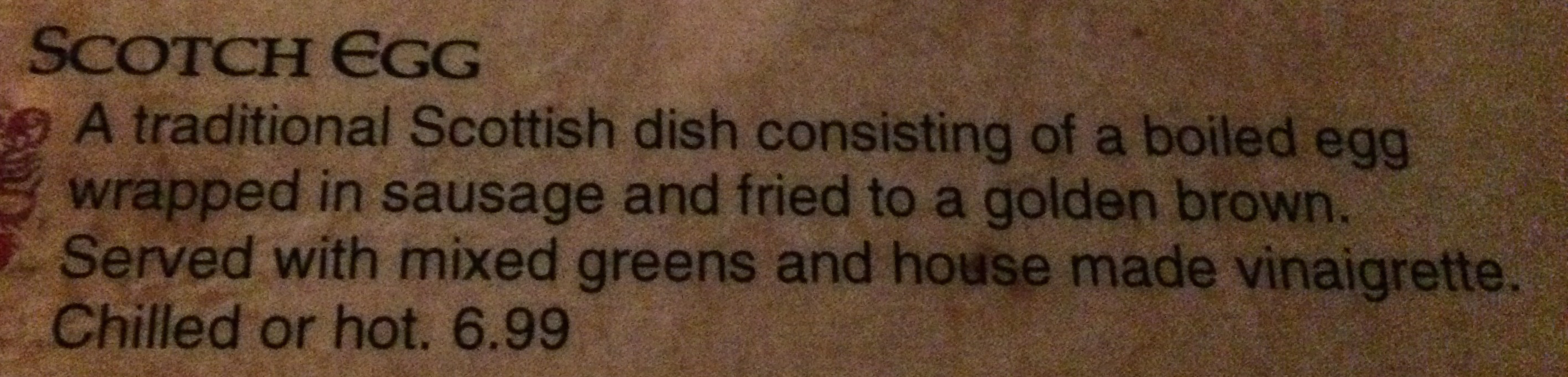This image features a horizontally oriented, very thin and short rectangle with a textured background of various blurred shades of brown, ranging from light tan to dark brown, giving it a smooth yet subtly grainy appearance. The background creates a tie-dye effect, blending multiple brown hues in an aesthetically pleasing manner. The main text, "SCOTCH EGG," is prominently displayed in a fancy black uppercase font at the center. To the left, there is a reddish-brown design featuring loops and intricate details, partially extending beyond the boundaries of the rectangle, adding an artistic touch. Beneath the "SCOTCH EGG" title, a detailed description in elegant black lettering reads: "A traditional Scottish dish consisting of a boiled egg wrapped in sausage and fried to a golden brown. Served with mixed greens and house-made vinaigrette, chilled or hot. $6.99."